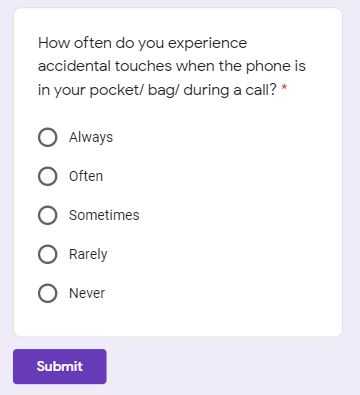The image features a light gray rectangle dominating the background. Within this rectangle, there is a centrally positioned white square featuring text in black font. The text poses the question, "How often do you experience accidental touches when the phone is in your pocket/bag/during a call?" accompanied by a small red asterisk indicating a required response.

Below the question, a series of selectable options are presented, each preceded by a circular button: 
1. Always
2. Often
3. Sometimes
4. Rarely
5. Never

These options are left-aligned and uniformly styled in black font, providing a clear and organized layout for user interaction. 

In the bottom left corner of the gray rectangle, outside the white square, there is a small purple rectangle. Within this purple rectangle, the word "SUBMIT" is bolded and displayed in white font, centered perfectly to catch the user's attention for finalizing their selection.